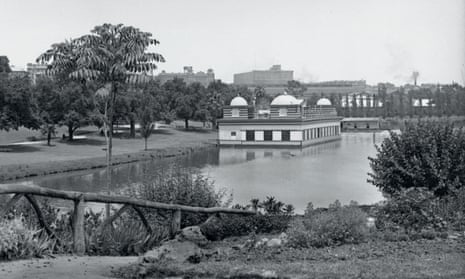This black and white photograph captures a still, daytime scene within a city, centering around a serene body of water. Dominating the image is a single-story boathouse, which features several small structures on its roof, including domed cabins. The water is calm, offering an undisturbed reflection of the overcast sky, which appears light and still. 

In the foreground, a wooden railing runs parallel to the water, bordered by short grasses and a bush located on the right side of the frame. The foreground also features patches of grass, some bushes, and a field, all showing signs of careful maintenance. The left side of the image reveals a tall tree with heavy foliage, situated on an embankment alongside more planted trees. 

In the background, the arches of a bridge and an out-of-focus building are visible, enhancing the urban setting of the scene. The photograph is devoid of people or boats, focusing solely on the tranquil waterscape and surrounding greenery.